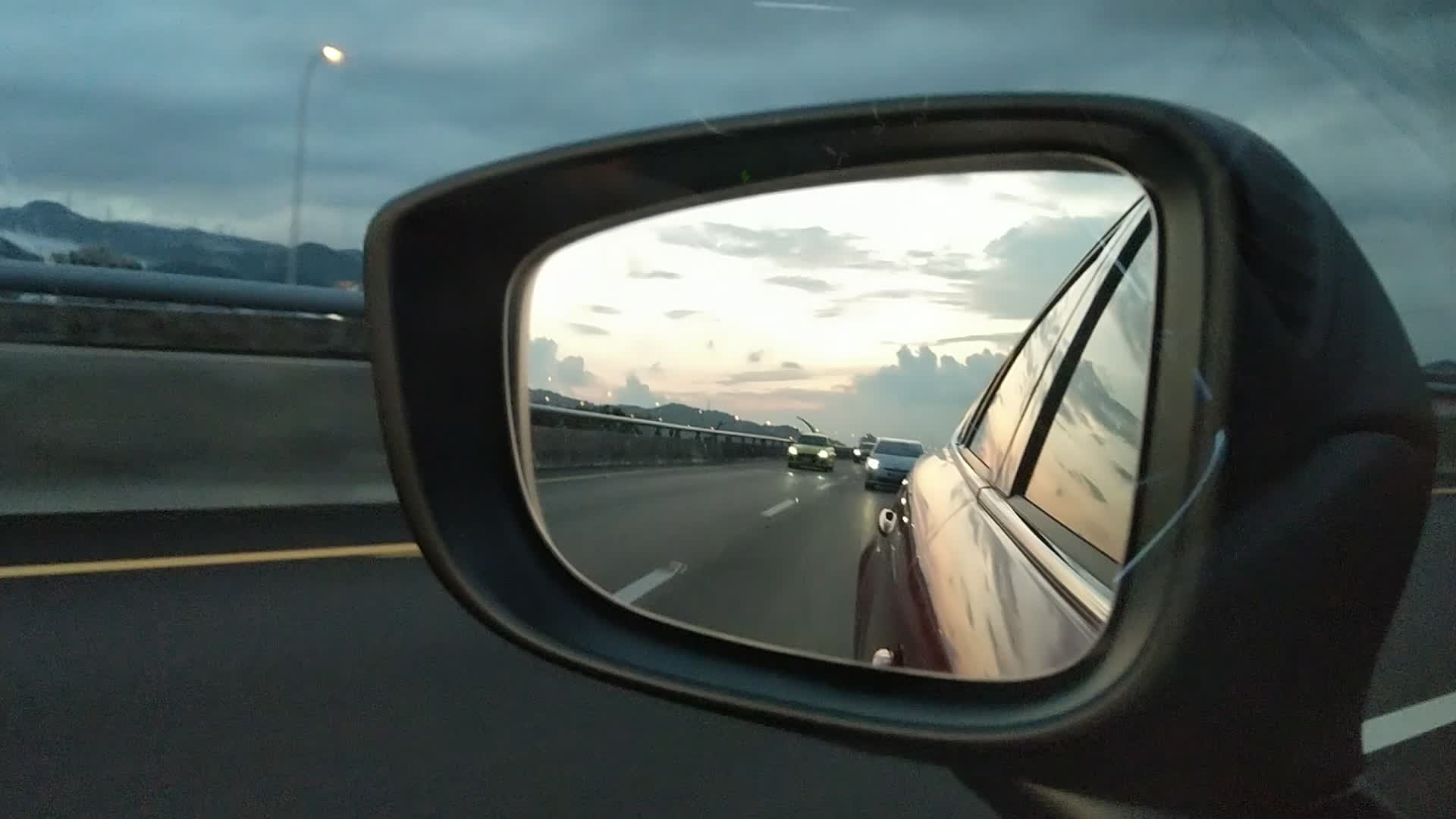A panoramic view features a vibrant blue sky adorned with scattered white clouds. A light pole stands tall with its light fixture visible at the top. In the foreground, a sturdy metal railing runs alongside a concrete divider. The ground consists of asphalt, marked with white lane lines. A side view mirror reflects the cloud-dappled sky and distant mountainous terrain. Approaching cars are visible with their headlights on, and the shiny side of the nearby car mirrors the serene sky, creating a captivating juxtaposition.